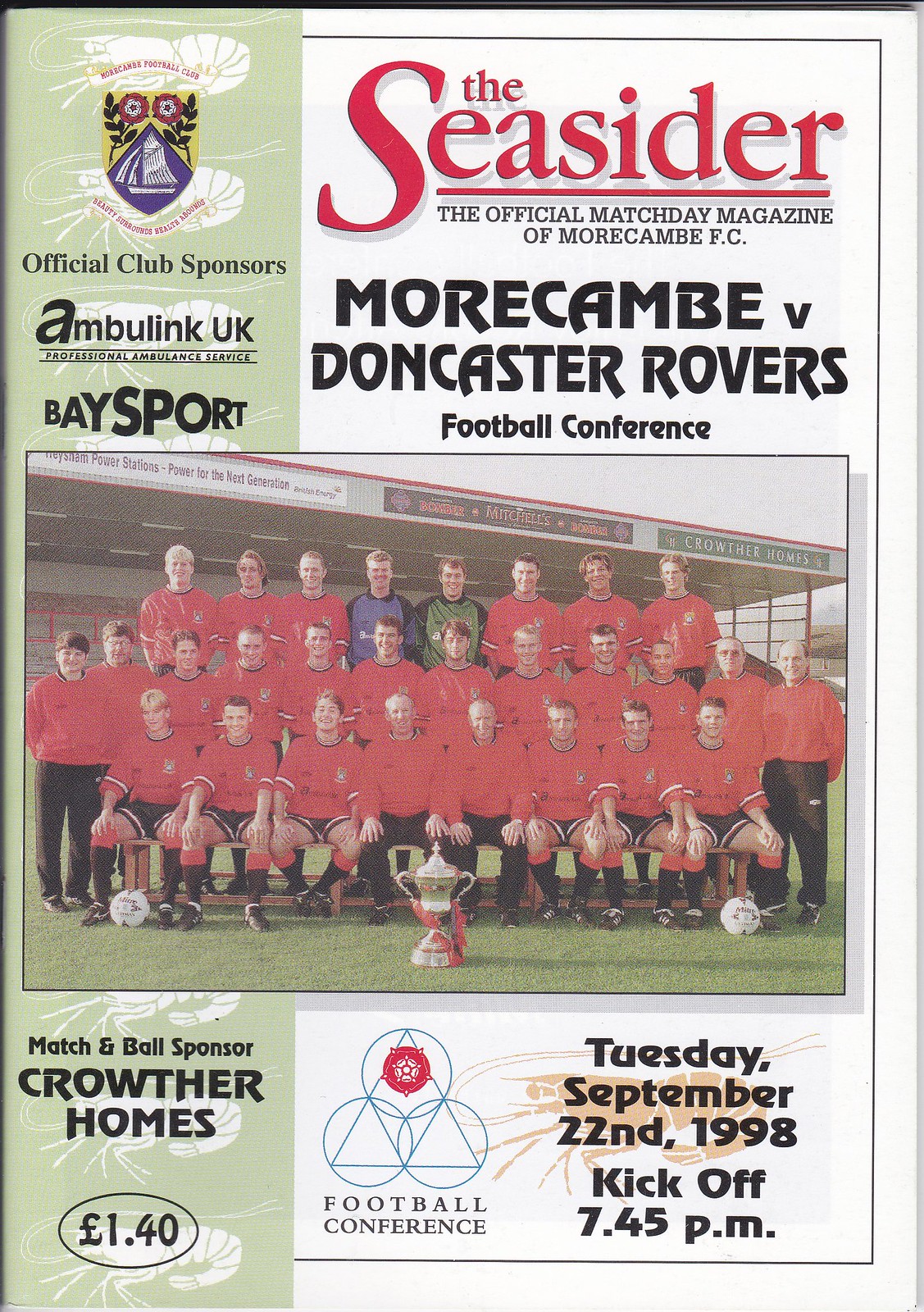The cover of the magazine "The Seasider", sporting a crisp white background with a pale green stripe running vertically down, prominently features the title in red ink, "The Seasider". Below, in black print, is the subtitle "The Official Match Day Magazine of Morecam F.C." and "Morecam V. Doncaster Rovers Football Conference" in bold black letters. On the left side, there is a white image of a shrimp adjacent to a yellow and blue shield adorned with flowers, which indicates "Official Club Sponsors: Ambulance UK, Baseball." 

In the center, a large color photograph captures a football team of men arranged in three rows: the first row seated, the second standing, and the third on an elevated stand. Most team members don red tops with black shorts, red and black socks, and sneakers, while two men in the back wear green and blue. The team is posed on a green grassy field, with a shiny vase-like trophy featuring handles prominently displayed at the front. White soccer balls are scattered around.

The cover also includes additional details such as "Tuesday September 22nd 1998, kickoff at 7:45 p.m." in black print below the image. On the far left, the price of "£1.40" is noted alongside the mention of "Match and Ball Sponsor Crowther Homes".